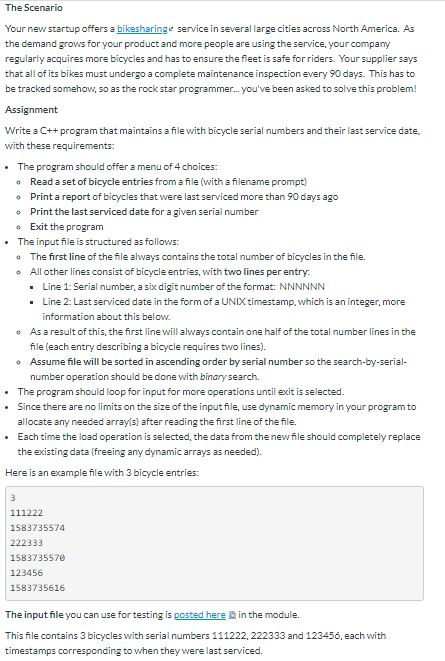This image contains text on a white background. At the top, there is a horizontal line followed by a bolded heading that reads "The Scenario." Beneath this heading, the text begins to describe the context: 

"Your new startup offers a bike-sharing service (with 'bike-sharing' highlighted in blue and underlined) in several large cities across North America. As the demand for your product grows and more people use the service, your company regularly requires more bicycles and must ensure the fleet is safe for riders. Your supplier mandates that all of its bikes undergo a complete maintenance inspection every 90 days. This needs to be tracked somehow."

The scenario then shifts to a task for the reader: 

"As the Rockstar programmer, you have been asked to solve this problem by writing a C++ program that maintains a file with bicycle serial numbers and their last service date. The program must meet the following requirements:
1. Offer a four-menu choice:
   - Read a set of bicycle entries
   - Print a report of bicycles that were last serviced
   - Print the last service date
   - Exit the program."

At the bottom of the image, within a square, it states: "Here is an example file with three bicycle entries. The input file you can use for testing is posted here in the module."

The caption of this image can be described in detail as follows:

An image with textual content on a white background, containing a scenario for a programming task. The heading, "The Scenario," is bolded, followed by a description of a bike-sharing service offered in North America, detailing the need for regular maintenance and tracking of bicycles. The text emphasizes the need for a C++ program to manage bicycle data, listing specific functionalities required of the program. Additionally, an example file and instructions for accessing a test input file are provided within a square at the bottom of the image.